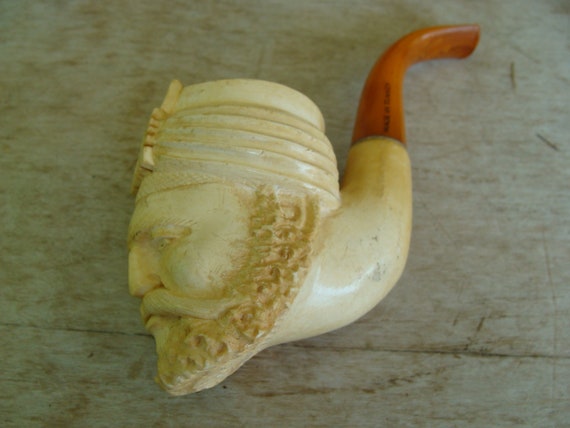This close-up image showcases a meticulously handcrafted smoking pipe, resting on a light wooden surface. The pipe is primarily composed of a white material, likely bone, tusk, or resin, and is artistically carved to depict the left profile of a man's head. The man, adorned with a turban or similar cloth headwear featuring an indiscernible front design, bears a full, dense curly beard and mustache that connect seamlessly with his hair. The man’s facial expression appears pensive or stern, accentuated by his downward gaze and sharp Roman-style nose.

The stem of the pipe, leading towards the mouthpiece, is made of a polished, reddish-brown wood, possibly light oak with a reddish tint, contrasting beautifully with the white of the carved head. It rises steeply from the intricately designed head and curves elegantly towards the user's mouth. The craftsmanship is evident in the detailed carving and the smooth, polished finish, making it a striking and functional piece of art.